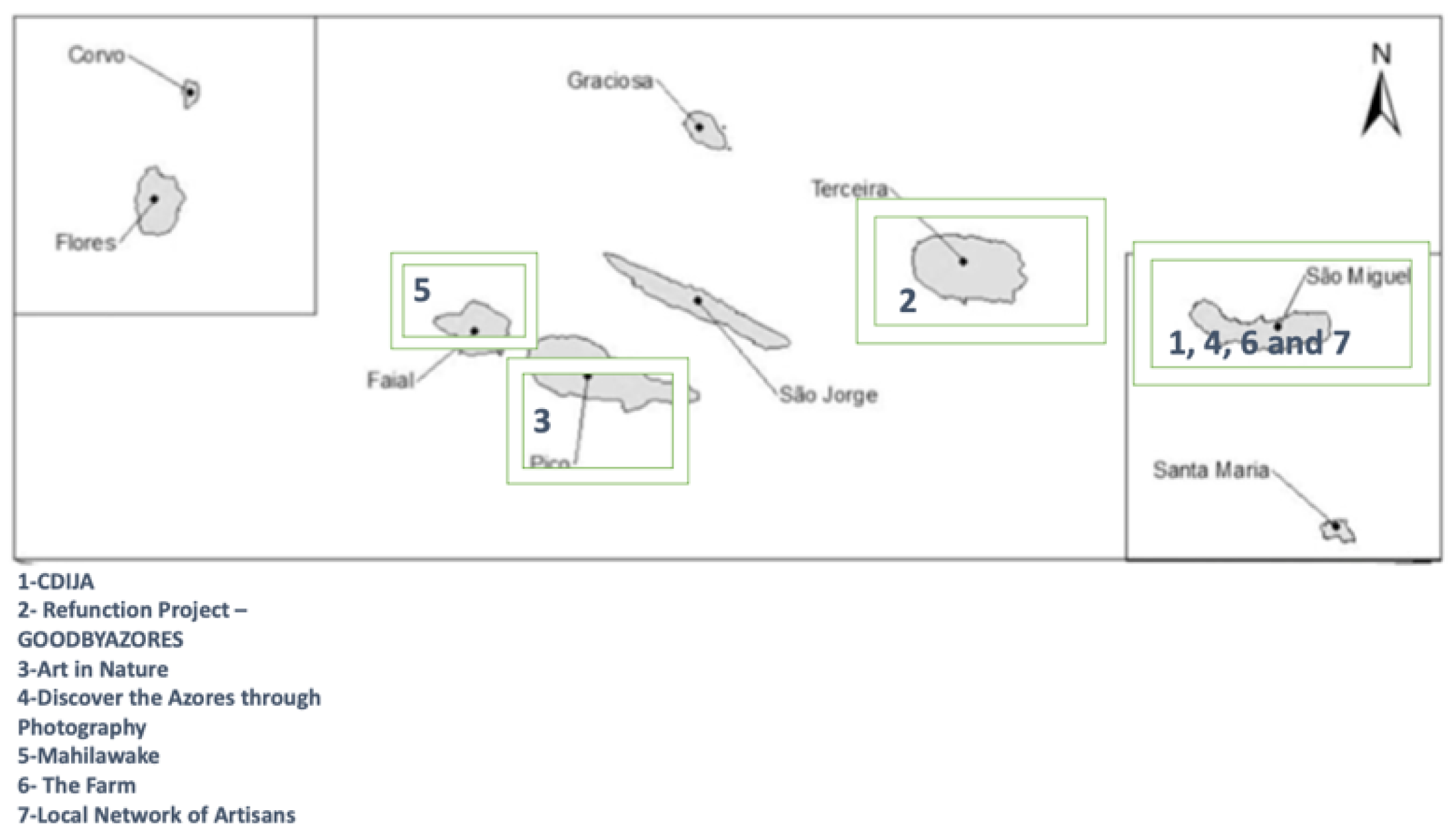The image is a black-and-white top-down map of several island shapes set against a pure white background. Each island is labeled with numbers or names, and there are annotations connected with lines that point to the light gray colored shapes. The map is oriented with a compass point in the top right corner indicating 'N' for north. In the top left-hand corner, a rectangle encloses illustrations of two islands with corresponding labels, while the bottom right-hand corner similarly highlights its own islands and annotations, connected by arrows.

In the bottom left corner of the map, there is a numbered legend arrayed vertically from 1 to 7. The items listed are: 1. C.D.I.J.A, 2. Refunction Project: Goodbye Azores, 3. Art in Nature, 4. Discovery in the Azores through Photography, 5. Mahilawaki, 6. The Farm, and 7. Local Network of Artisans. Additionally, several islands are surrounded by green rectangles, some of which do not fully cover the islands but are offset somewhat. The style of the illustration is infographic with a detailed emphasis on naming and labeling, capturing both the geographical layout and thematic projects associated with the islands.